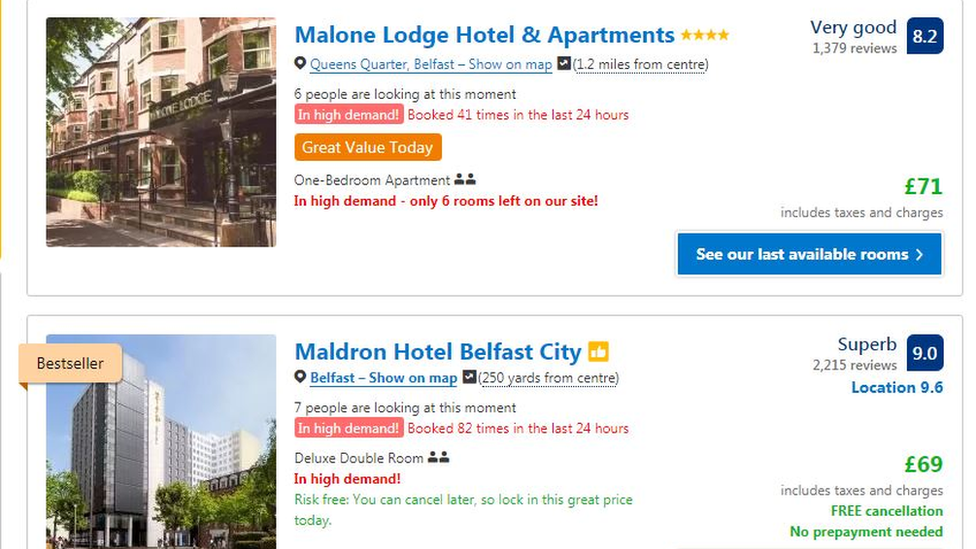A screen capture displays two accommodation options, each showcasing high demand. 

The first option is the Malone Lodge Hotel and Apartments located in Queens Quarter, Belfast. It features a one-bedroom apartment available for £71 per night. The listing highlights its popularity with six people currently viewing the offer and 41 bookings made in the last 24 hours.

The second option is the Maldron Hotel in Belfast City, recognizable by its high-rise structure. This selection is labeled as a "Bestseller" with a nightly rate of £69. It is also experiencing high demand, with seven active viewers and 82 bookings within the last 24 hours.